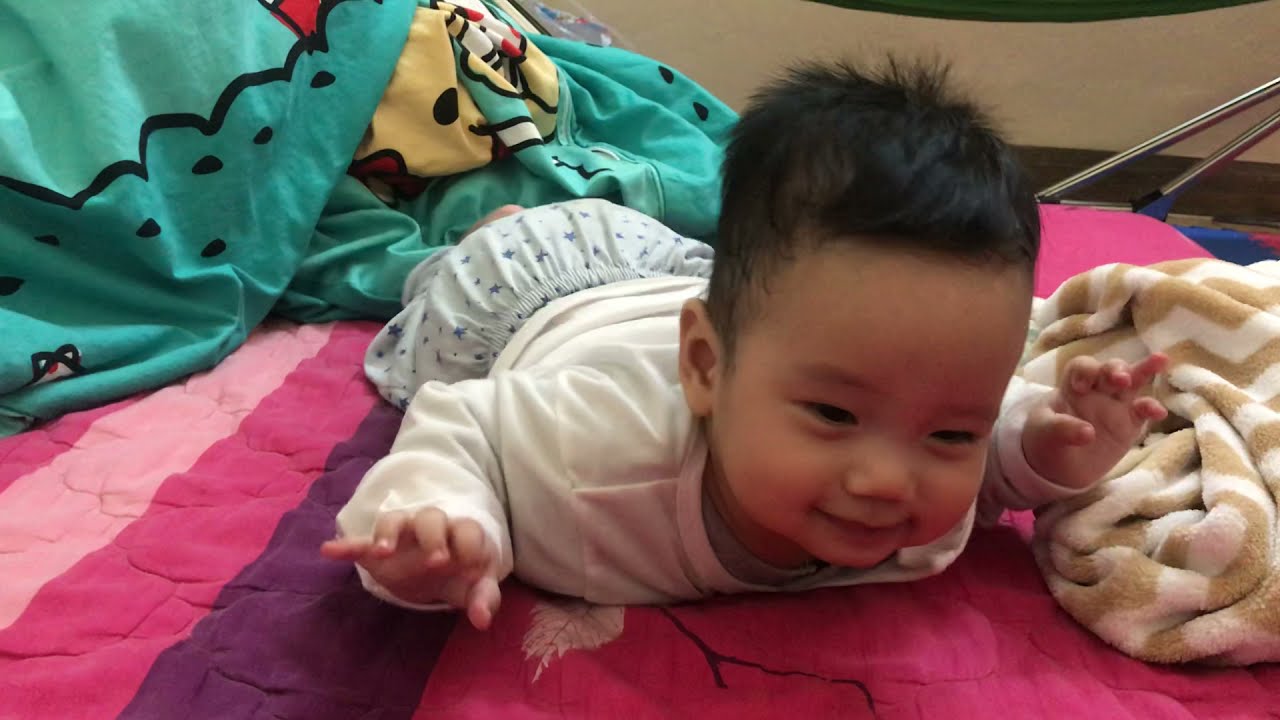The image depicts a smiling toddler of Asian descent, likely around one year old, lying on their stomach in a planking position. The baby, with short, slightly spiky black hair, is centrally positioned and occupies about half of the image. They are wearing a long-sleeved white shirt and blue shorts adorned with stars. The toddler's head is lifted, and their hands are raised off a pink blanket that features multiple pink stripes, a dark purple stripe, and a white leaf design. 

Directly behind the child, there is another crumpled blanket that is primarily green with a scalloped black border, incorporating some muted lighter shades and black dots. On the right-hand side of the image, near the baby's left hand, is another folded blanket with white and light brown zigzag patterns. All elements suggest that the scene is indoors. The toddler's joyful expression and playful pose contribute to a warm, lively atmosphere.